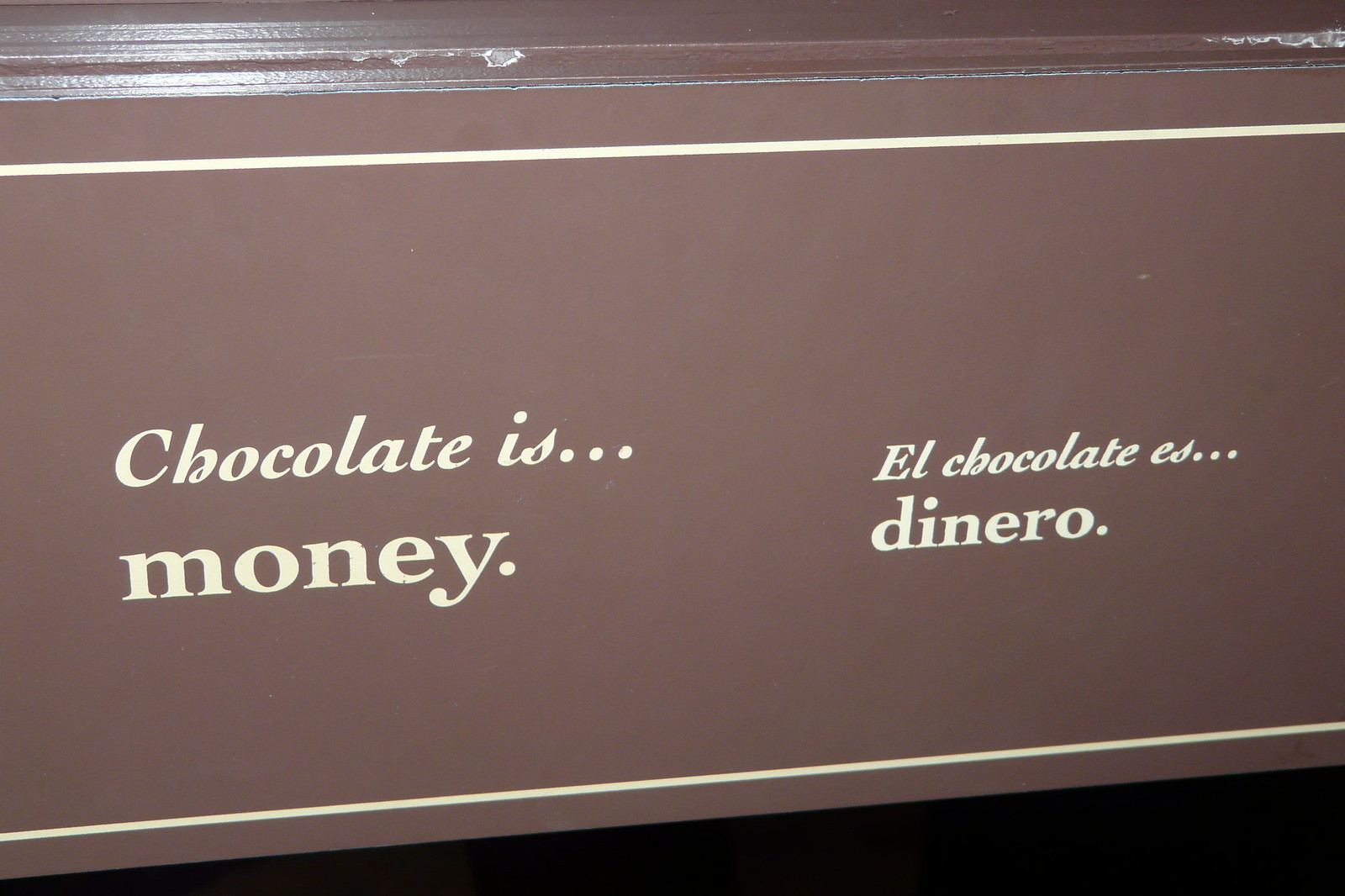The image depicts a light brown wooden fixture, likely part of a sign or a permanent installation on a wall or counter. The wood shows signs of wear, particularly at the top left and right corners, where the paint is scratched and worn off. The top and bottom edges of the wood are bordered by cream-colored lines. In the center, the sign features a bilingual message in the same cream hue: on the left, it reads "chocolate is... money," and on the right, "el chocolate es... dinero." This suggests a playful equivalence between chocolate and money, both in English and Spanish.